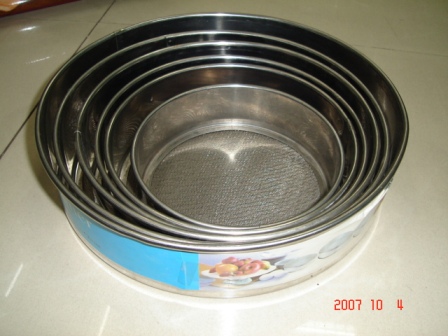This detailed photograph, taken on October 4th, 2007, shows a set of stacked metal sieves positioned on a white, tiled countertop. The sieves, with silver steel rims, are meticulously arranged from the largest on the outside to the smallest at the center, each fitting snugly within the other. The smallest sieve at the center reveals a fine metal mesh and a reflective bottom. A prominent blue label adorned with an image of fruit decorates the front of the outermost sieve. In the lower right corner of the image, the date "2007-10-4" is displayed in red letters, adding a timestamp to this perfectly organized kitchenware arrangement.